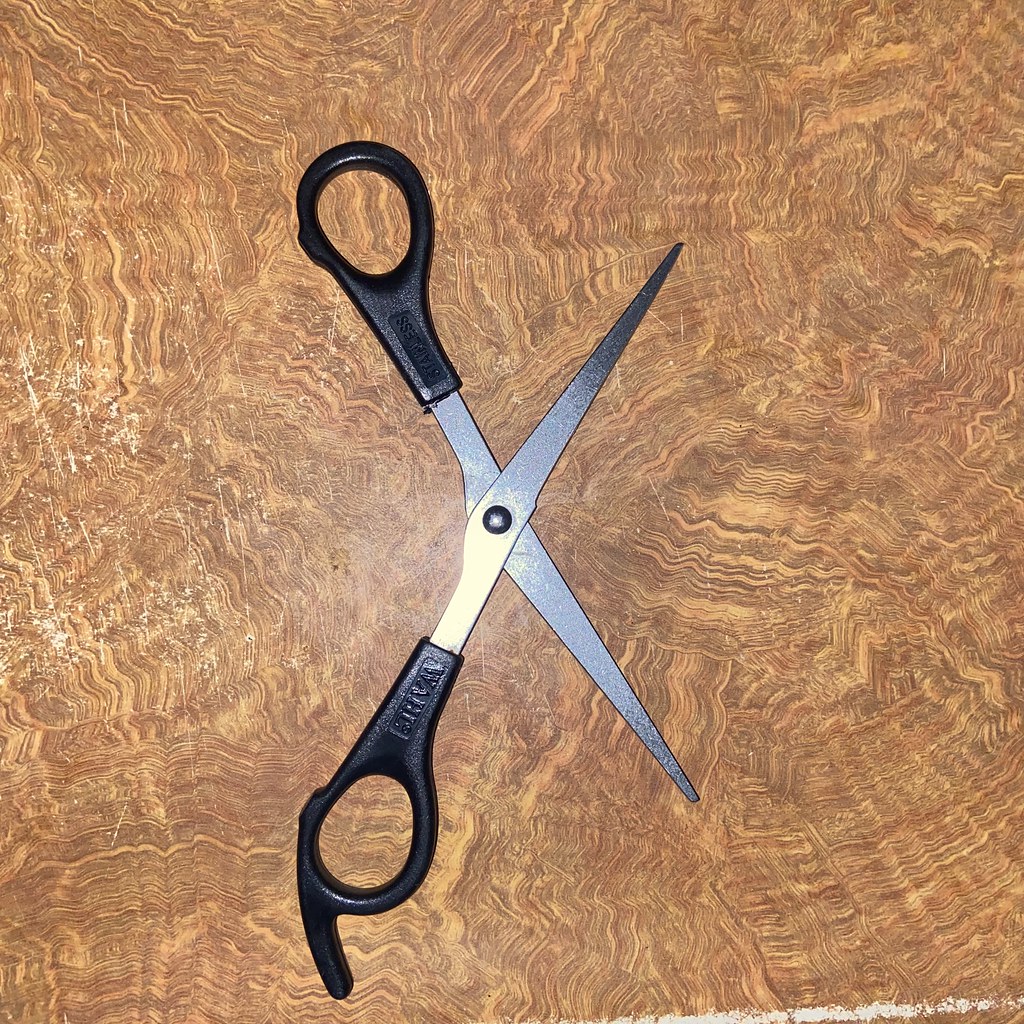This image portrays a pair of scissors resting open on a wooden tabletop with a striking burl wood pattern, although some suspect it might be a textured vinyl imitation. The wood surface displays noticeable grain patterns and wear, including a white scratch or mark in the bottom right corner. The scissors are silver, likely stainless steel, and feature black handles made possibly of plastic, rubber, or nylon. One handle has a distinctive elongated piece of plastic curving around the loop, held together by a black painted round circle. Although some markings are visible on the scissors, the brand name is obscure, possibly reading "W-A-R-E." The scissors’ sharp blades point to the right, lying amid the intricate swirls of the wood grain, and hints of surface damage indicative of wear or past exposure to moisture.